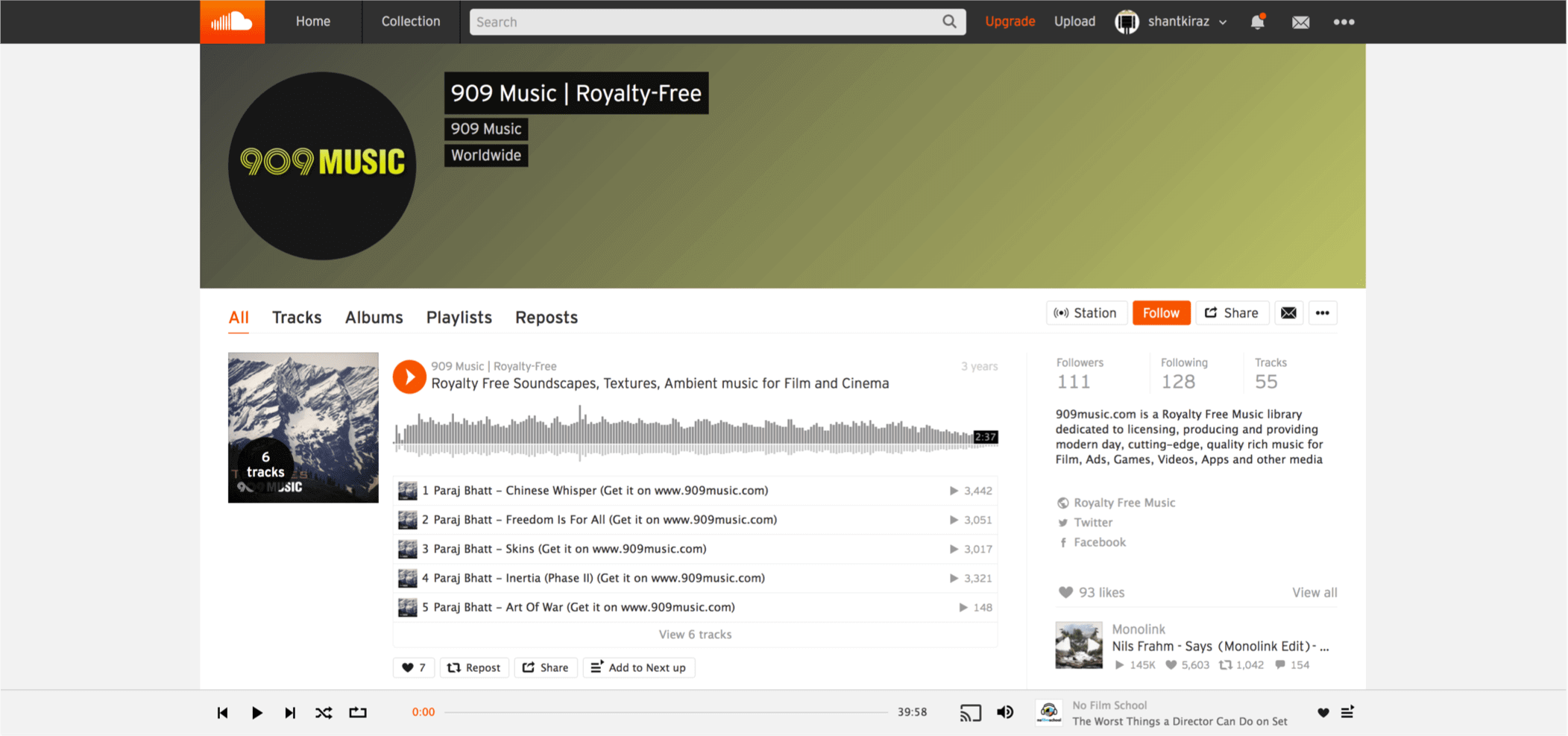This is a screenshot of the SoundCloud website, showing a specific artist's page. In the top left corner, the SoundCloud logo is prominently displayed; it features a cloud design, half of which is made up of segmented lines. The logo is white, set against an orange background. The top menu bar includes buttons for "Home" and "Collection."

Adjacent to the menu bar, the search bar is visible, featuring options for "Upgrade" and "Upload," along with a user profile drop-down menu. Just below this, a black header bar displays the text "909 Music Royalty Free." To the left of this header, there is a circular profile picture with a black background and yellow text that reads "909 Music."

Beneath the profile picture, several navigation tabs are available, including options for "All Tracks," "Albums," "Playlists," and "Reposts." Below these tabs, an audio player is integrated into the page, providing a seamless listening experience.